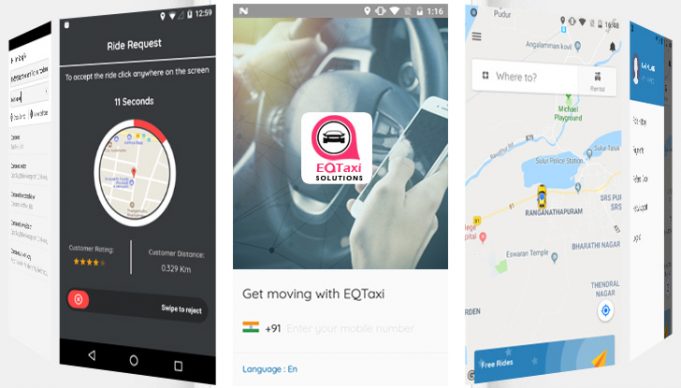This image features a carousel arrangement of four to five screenshots showcasing an EQTaxi mobile application. Prominently, the screenshots include interactive text prompts such as "ride requests," directing users to "accept the ride," and highlighting a unique "click anywhere on the screen" feature, all within an 11-second timeframe. The brand's tagline, "Get moving with EQTaxi," and a "Where to?" input field are also visible, underlining the app's user-friendly navigation.

A centrally-placed screenshot features an Indian flag and confirms the language setting as English. To the left, additional screenshots reveal a grey background, complemented by navigation buttons at the bottom, emphasizing the app's intuitive design. The images collectively demonstrate a diverse color palette including black, white, red, blue, and orange, with a consistent status bar present across all screenshots. This detailed visual representation underscores EQTaxi's mission to streamline user experience and enhance accessibility.